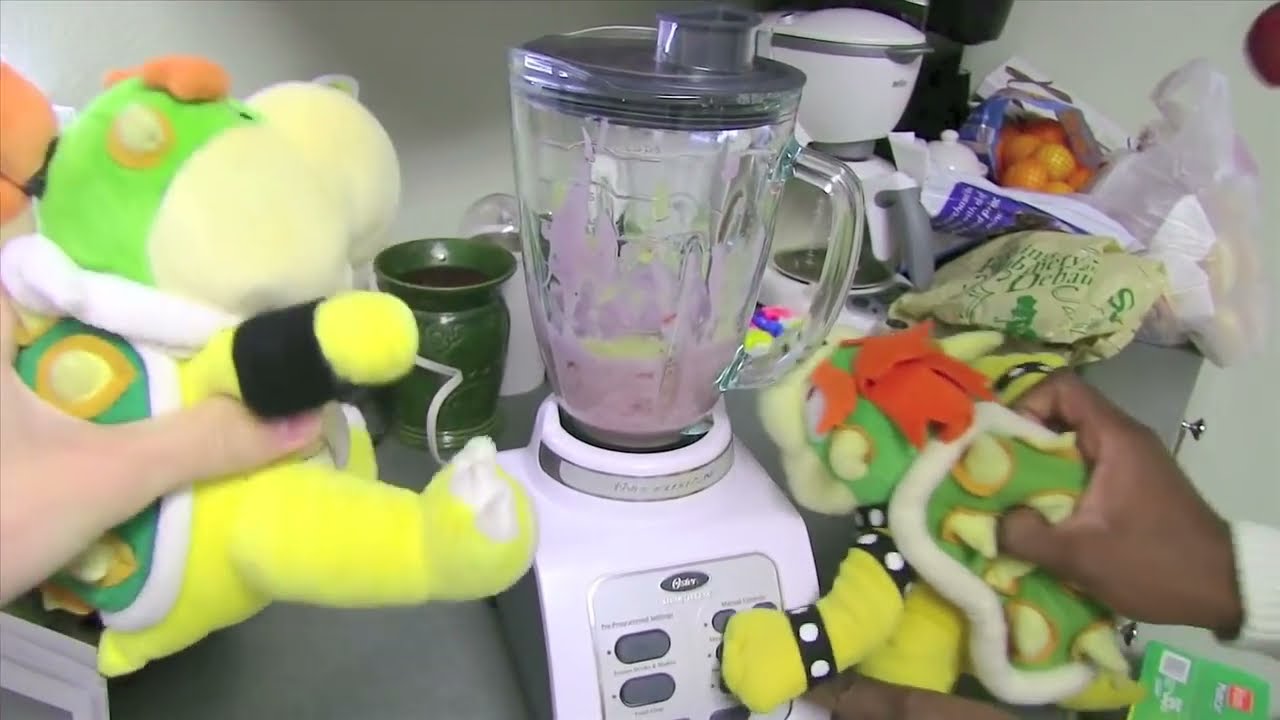In a bustling kitchen scene, a white and gray Oster blender, mid-process with a purple liquid inside, stands prominently at the center of a cluttered counter. To the left, a person with a peach complexion holds a small Bowser stuffed animal, while on the right, a person with caramel-colored skin holds a larger Bowser plush toy. Behind the blender, a dark green vase, a white coffee pot, a bag of oranges, and several plastic bags create a backdrop of everyday kitchen chaos. The vivid colors of the Bowser toys—with their yellow skin, red and green accents, black wristbands, and spiky shells—contrast with the disarrayed counter, suggesting an impromptu, perhaps humorous scene involving the stuffed animals interacting with the blending process, reminiscent of a playful moment caught in the middle of a homemade video or family activity.